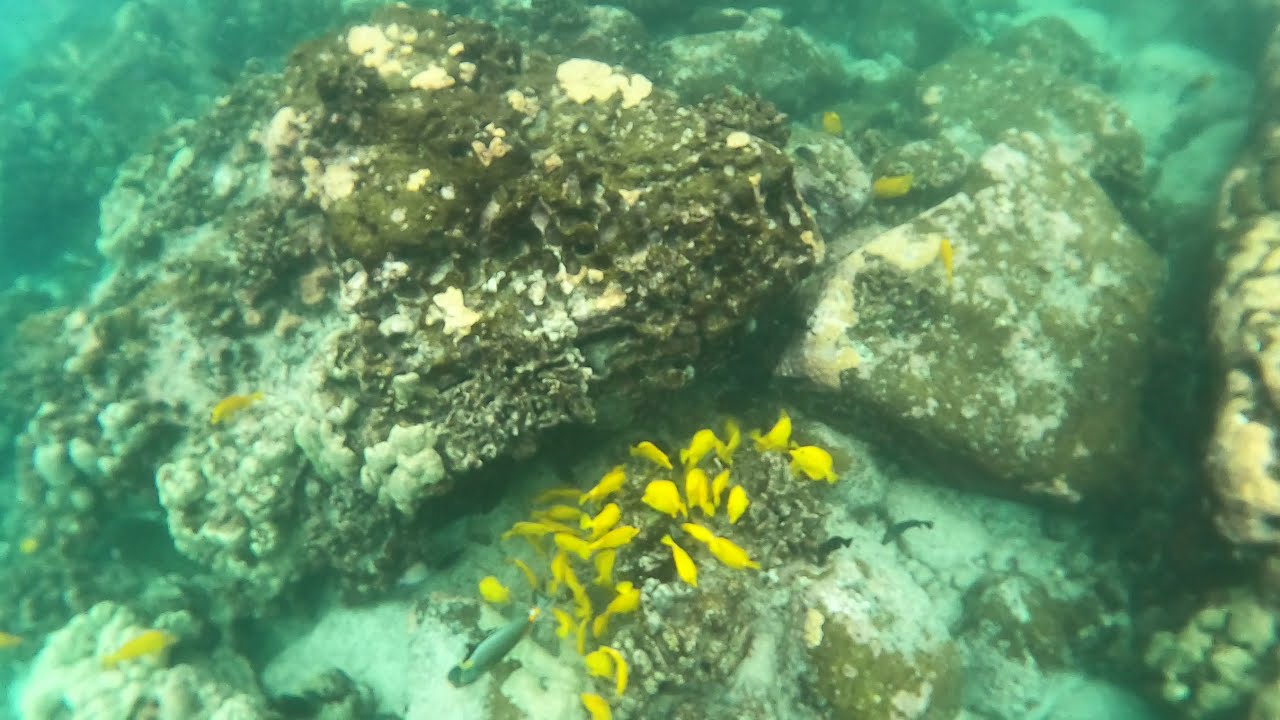This horizontally aligned rectangular image captures a dynamic underwater scene. Dominating the frame is a diverse array of large boulders at the bottom, worn by water and covered in colorful growths, including coral and algae. The boulders exhibit vibrant hues of green, brown, and white. Amidst this rocky seabed, a school of small, bright yellow fish is vividly featured, swimming in various directions. While most of these yellow fish remain clustered in the center of the image, a few venture away from the group. Additionally, there are a couple of other fish species visible: a longer silver fish and smaller dark, likely black fish, contributing to the sense of aquatic diversity. The water itself has a medium clarity, with a predominant green tint that appears slightly clearer in some areas. This verdant hue tends to blur the extremities of the photograph, adding to the immersive underwater atmosphere.